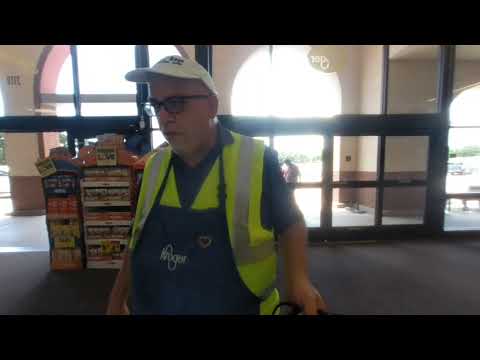The photograph depicts an older white man, a grocery store worker, prominently positioned in the foreground. He is attired in a blue polo shirt beneath a green safety vest, a white baseball cap, and black glasses. Over his shirt, he wears a blue apron emblazoned with the word “Kroger.” The worker is looking to the left and holding an unidentified object, its handle visible.

In the background, the lobby of the Kroger store is visible, featuring a carpeted floor and two sets of automatic double glass doors, one of which is open. Through these doors, a sidewalk and a white pillar with dark brown edges are partially visible. Inside the entrance, to the left, there is a colorful display containing red, blue, and yellow items, although the details are somewhat blurry. Additionally, a customer in a white shirt can be seen walking towards the store, looking down at the ground.